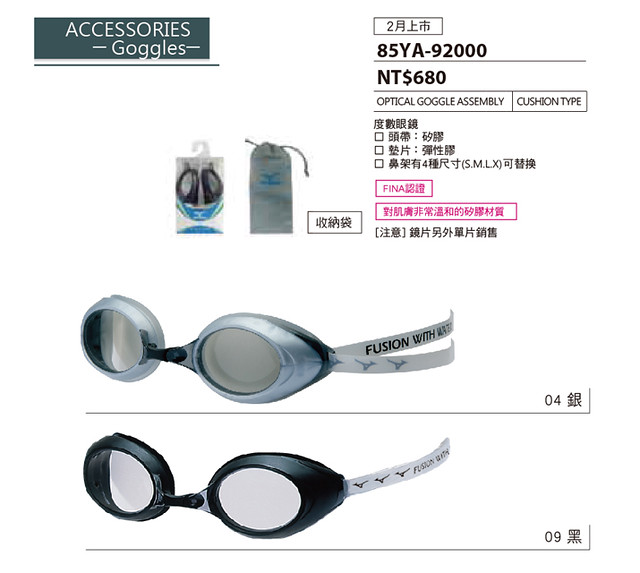The image is an advertisement for optical goggle assembly, cushion-type eyewear, displayed on a website. The website banner at the top left corner displays the words "Accessories" and "Goggles" against a grayish background. The ad features two sets of goggles: one with black rims and white stripes around the lenses, and another with silver rims and white straps, where one strap is partially readable and says "fusion with." Both sets of goggles are individually packed in plastic packaging with hang tabs for display in stores. The packaging is complemented by a silver net bag for storage, adorned with a small blue emblem. Additionally, black plastic accessories in a clear bag are shown, though their specific purpose is unclear. Positioned on the top right is model number A5YA-922000, and the price is listed as NT$680. There is also textual information in an Asian language providing further details about the product.